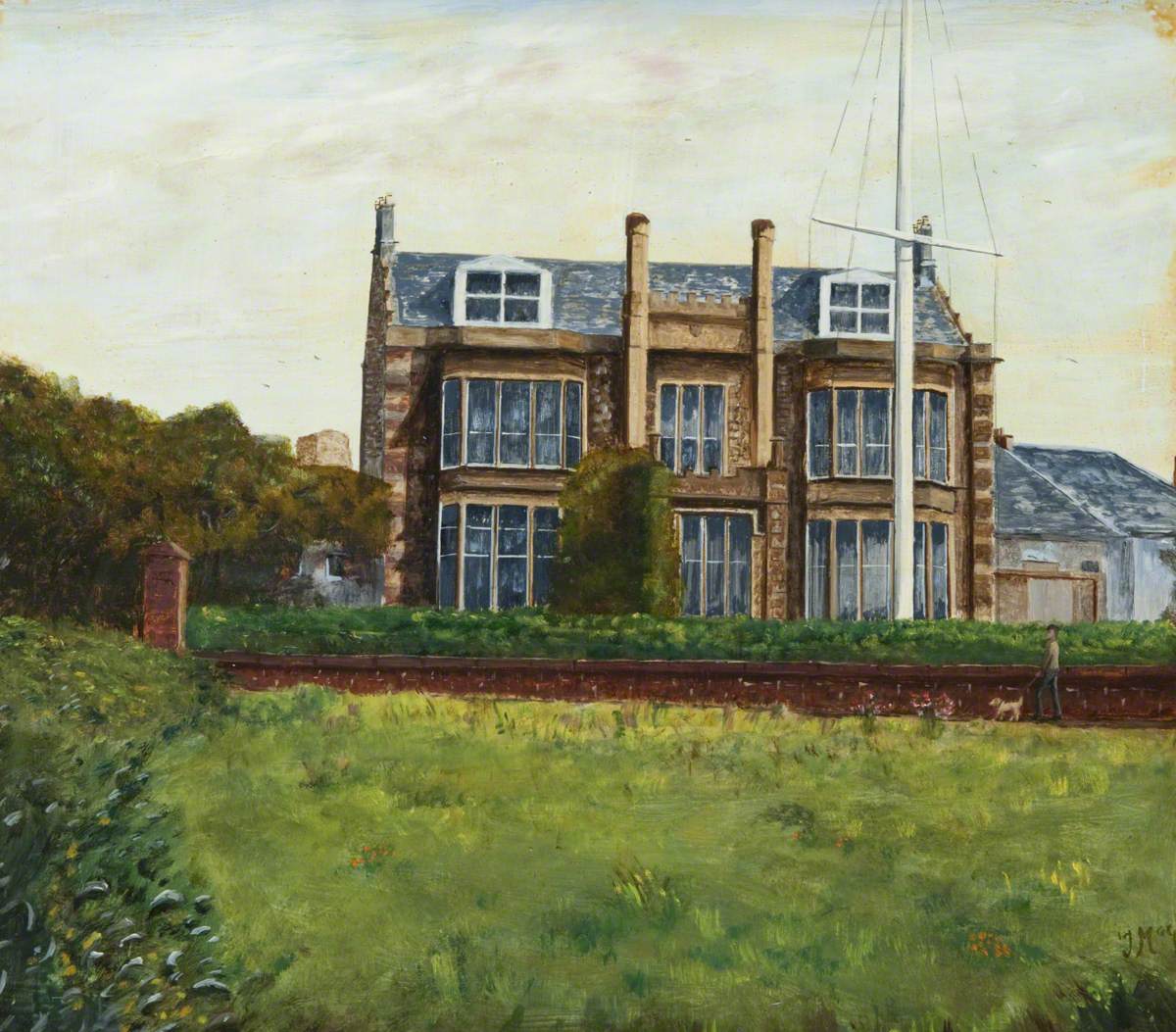This vertically oriented painting showcases a two-story home constructed from dark brown brick, prominently featuring extensive window sections. Each side of the house, both in the front and the center, displays groups of four vertical rectangular windows arranged directly above one another across both floors. Adding architectural intrigue, the blue roof boasts a unique slanting design, rising from the front to a peak before descending to the back. It's adorned with white dots and crowning windows on either side of the roof's base.

The house is nestled amid a lush environment filled with green trees and grass, under a very pale light blue sky, suggestive of a tranquil daytime scene. Complementing this pastoral setting, there appears to be a boat with a distinctive sail and mast in the foreground, hinting at the house's proximity to water. An additional building is positioned to the right, enhancing the composition's balance. The painting employs a vivid palette of brown, light brown, tan, white, various shades of green, yellow, beige, and black, vividly capturing the idyllic setting.